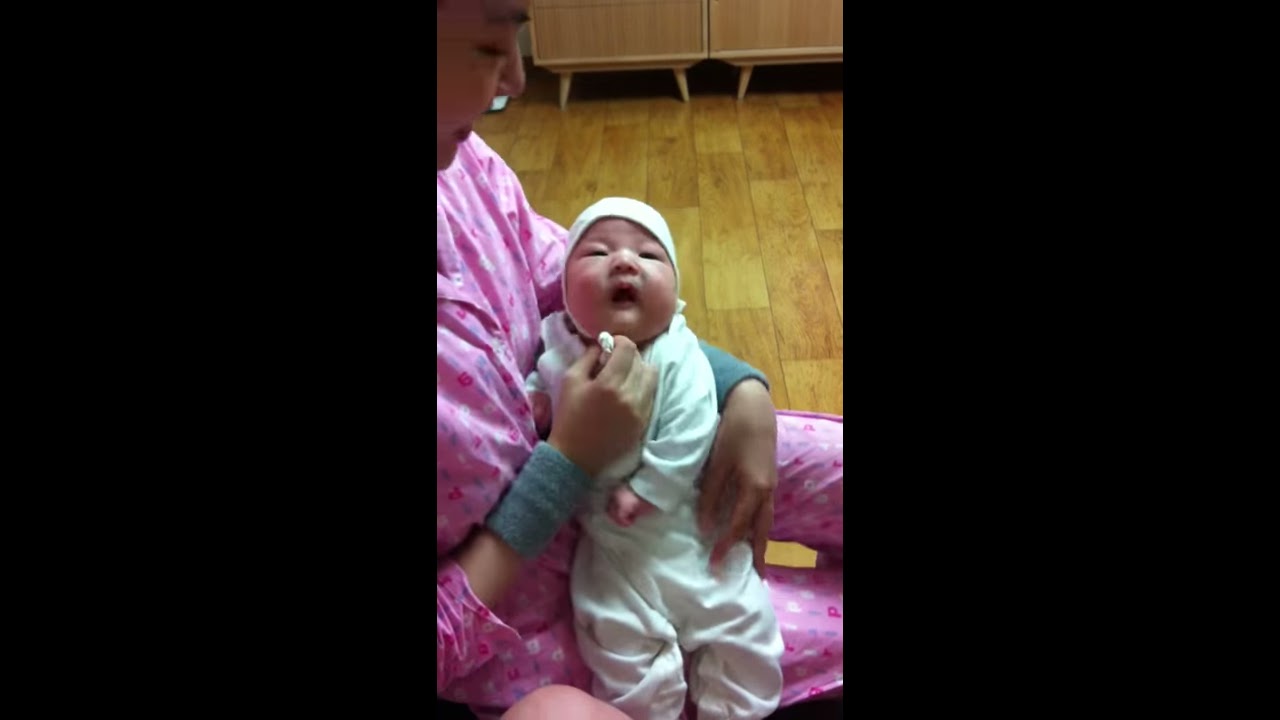In this vertical cell phone image, a woman, likely the mother, is tenderly caring for a very young, possibly newborn, baby. The mother is dressed in a pink outfit, resembling either pajamas or a hospital gown, and she has large, fluffy wristbands around her wrists. She is seated, holding the baby in her lap with her left arm supporting the baby's back. The baby, swaddled in a white onesie and wearing a matching hat, is facing the camera with an open mouth and a serene, almost goofy expression. Using her right hand, the mother appears to be offering the baby a pacifier. The scene is set indoors, lit by fluorescent lighting, with a hardwood floor visible beneath them. In the background, partially visible, are the feet of a couple of cabinets framing the scene. The warm, nurturing atmosphere suggests this may be a moment shortly after the baby's birth, possibly still in the hospital.